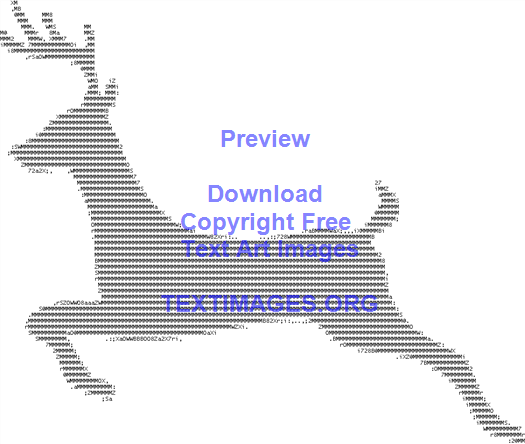The image features a computer-generated depiction of a black buck, seen in profile, prancing against a stark white background. The deer, distinguished by its full rack of antlers, appears as though it is created using an intricate repetition of small symbols or characters, which blend together to form its shape. Blue text overlays the image, reading "preview, download, copyright free, text art images, textimages.org." This text, located predominantly in the middle and bottom sections of the image, is notably difficult to read due to its diminutive size and the complex artistry of the image. The deer’s front legs are raised, capturing a sense of motion and vitality in this meticulously crafted digital artwork.